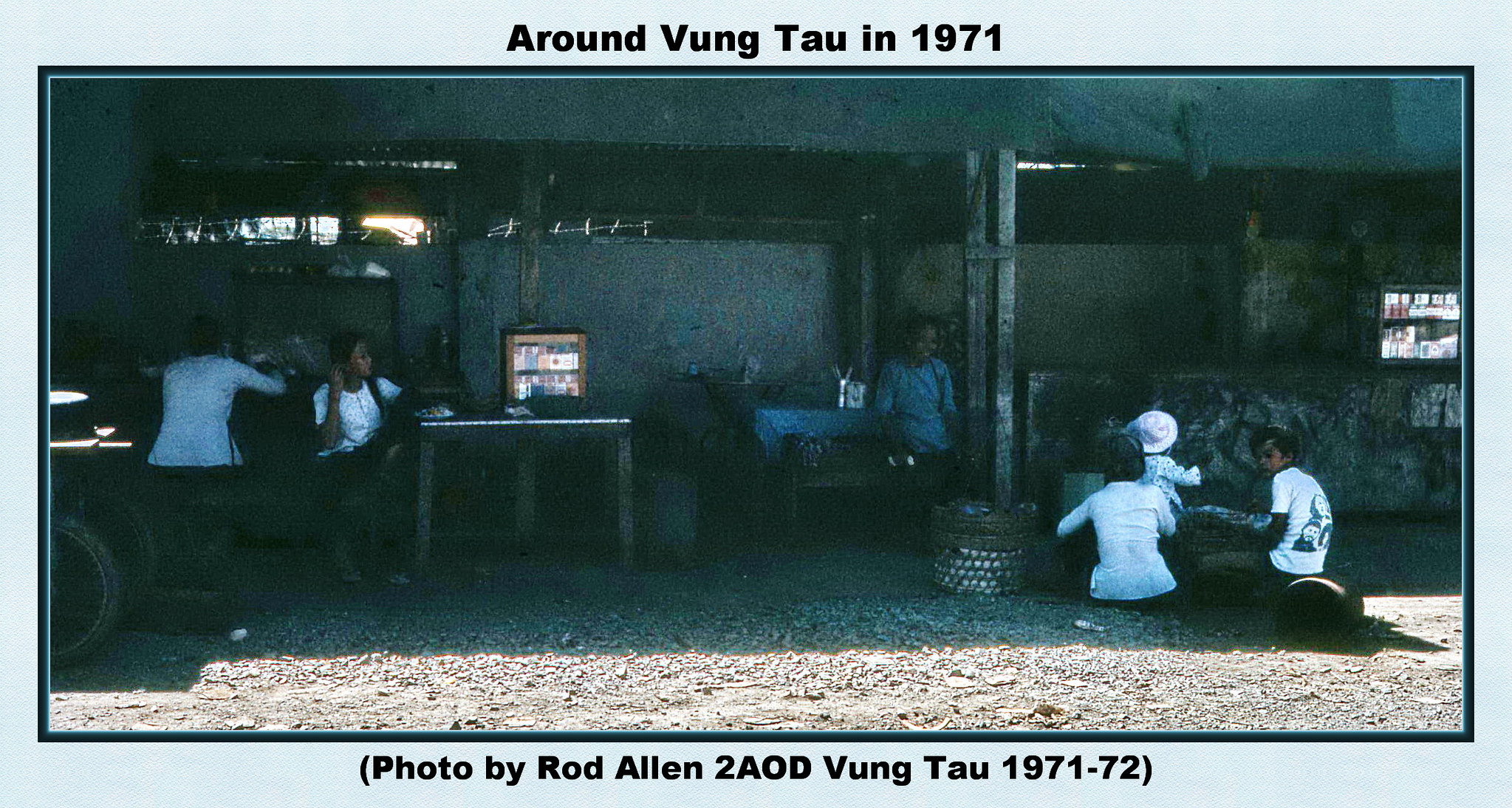The color photograph, framed within a light blue border that itself is enclosed by an inner black border, captures a moment Around Vung Tau in 1971, as indicated by the black font on the top of the blue border. The bottom blue border provides additional context with the inscription, "Photo by Rod Allen, 2AOD, Vung Tau, 1971-72." The image features six people in an outdoor setting that appears to be part of a home or a similar informal environment. 

On the right side of the photograph, three children are seated on the ground near a smiling woman who is also seated and facing them. To the left, two individuals are seated; one has their back turned to the camera, while the other faces the camera, looking to their left. They are near tables holding various items. The ground is a mix of dirt and rocks, suggesting a rugged, unpaved area. In the background, a solid concrete wall and flat concrete ceiling, supported by pillars, create a shaded area where people are gathered. There's also a concrete counter with a refrigeration unit behind it, sporting a clear glass door that reveals various boxes and bottles inside.